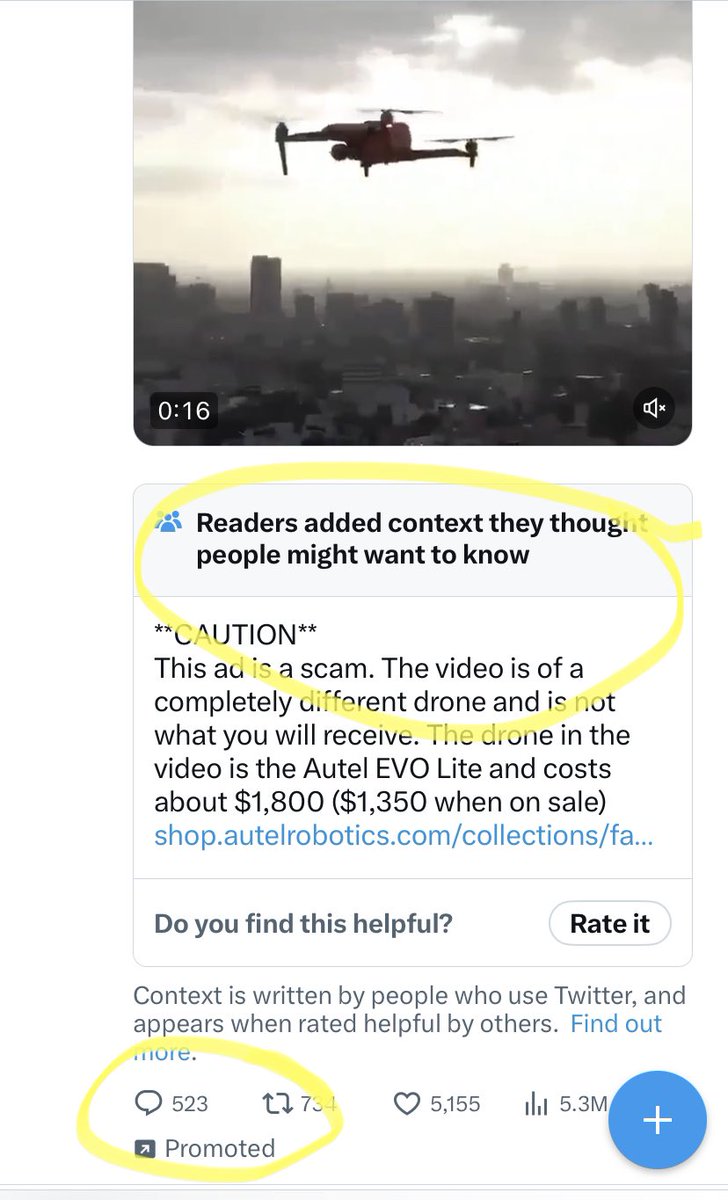This screenshot captures a promoted ad on Twitter, featuring various interactive elements and a high engagement rate. At the top, there's a video displaying a drone flying over a foggy, brownish-hued cityscape, with clouds indicating the early hours of the day. The video duration is 16 seconds, and a muted audio icon is at the bottom right corner, marked by an "X" over the speaker symbol.

Below the video, social interaction buttons are present: a comment bubble on the bottom left, a retweet button in the center, and a heart-shaped like button on the right. The post has accumulated significant engagement, with 523 comments, 734 retweets, and 5,155 likes. The view count stands impressively at 5.3 million.

Prominent yellow circles highlight important information. The central circle indicates that readers have added context to the ad, clarifying that "Caution: This ad is a scam." This warning serves as a critical alert for viewers to be wary of the ad's legitimacy.